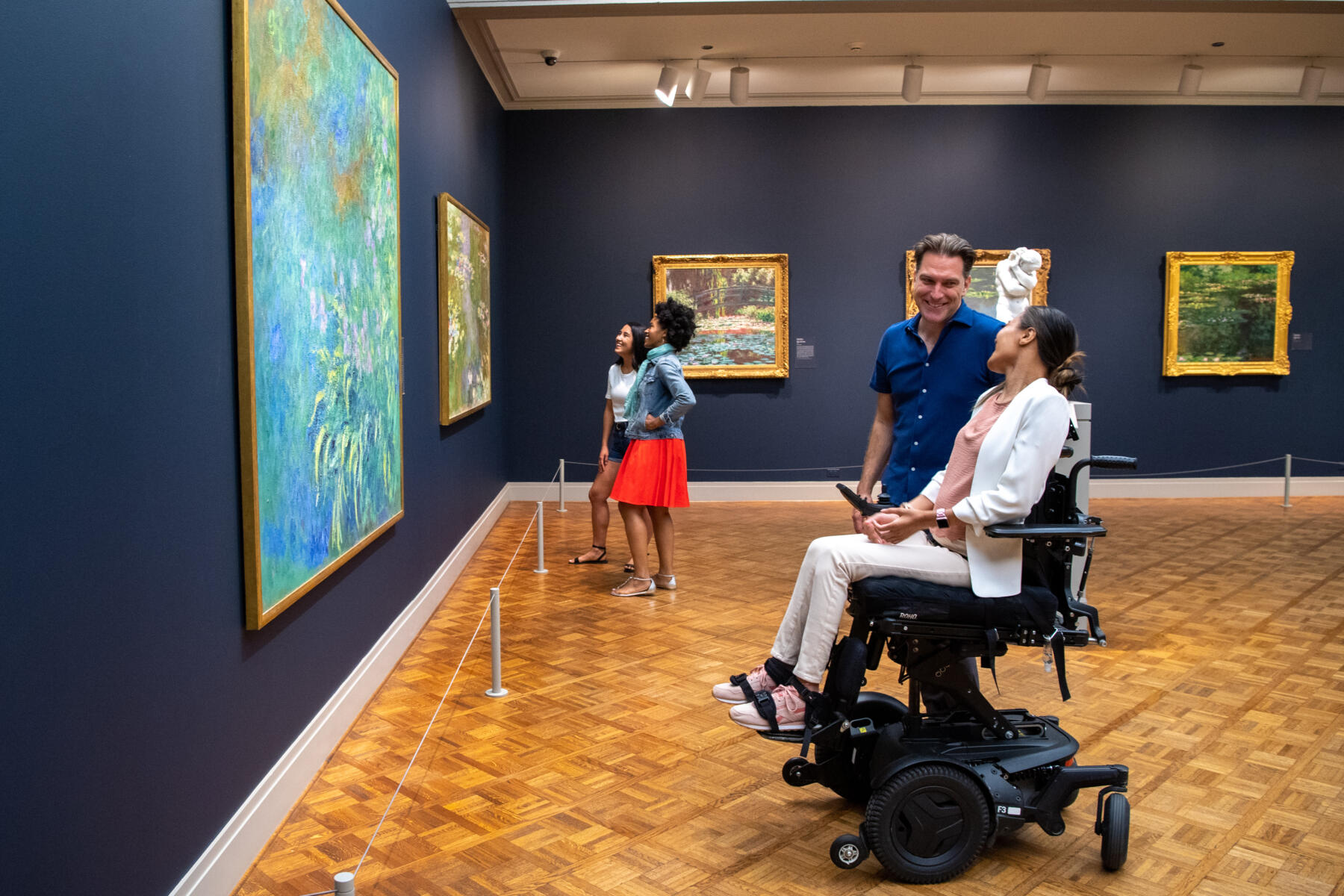This detailed photograph captures an intimate moment inside a navy blue-walled museum, featuring a blend of Impressionist art, including five paintings and a marble statue, all adorned in gilded gold frames. The spotlight-illuminated exhibit is cordoned off by white stanchions linked with sleek ropes, ensuring viewers maintain a respectful distance. The floor showcases a light tan wood parquet pattern, adding elegance to the gallery's ambiance. 

In the foreground, a woman with dark hair and pale skin sits in a motorized wheelchair, clad in white pants, a white jacket, and a rose-colored blouse, engaging warmly with a man in a dark blue shirt standing beside her. Both share a smiling exchange, adding a poignant, personal touch to the scene. 

Further back, two younger women are engrossed in the artwork. One, dressed in a red skirt and blue denim jacket with dark hair and skin, stands beside another woman wearing dark shorts and a white top. Both appear captivated by a smaller piece displayed on the left wall, each detail reflecting the enriching experience of their museum visit.